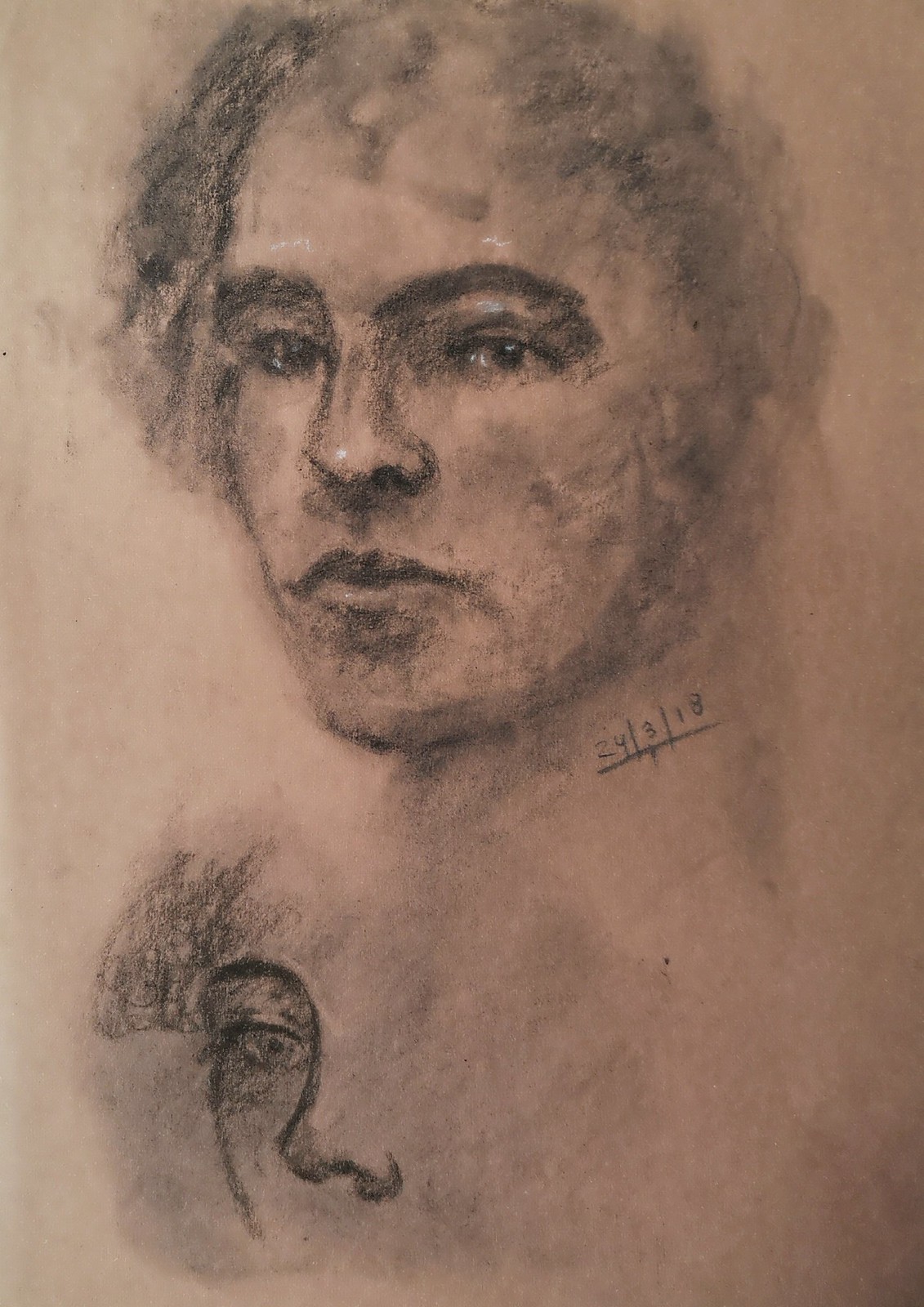A detailed and cleaned-up version of the given caption could be:

---

This artwork, dated 24/03/2018, appears to be a historical portrait, potentially of a figure like Mozart or another prominent figure from the past. The date notation suggests it is of English origin. The portrayal features a man with prominent, heavy eyebrows and thinning, curly hair, receding significantly at the top, with small waves of hair cascading down. There's a somewhat confusing element included in the image that resembles a finger, adding an enigmatic touch to the overall composition.

---

This caption provides clear and concise information while ensuring detail and avoiding redundancy.